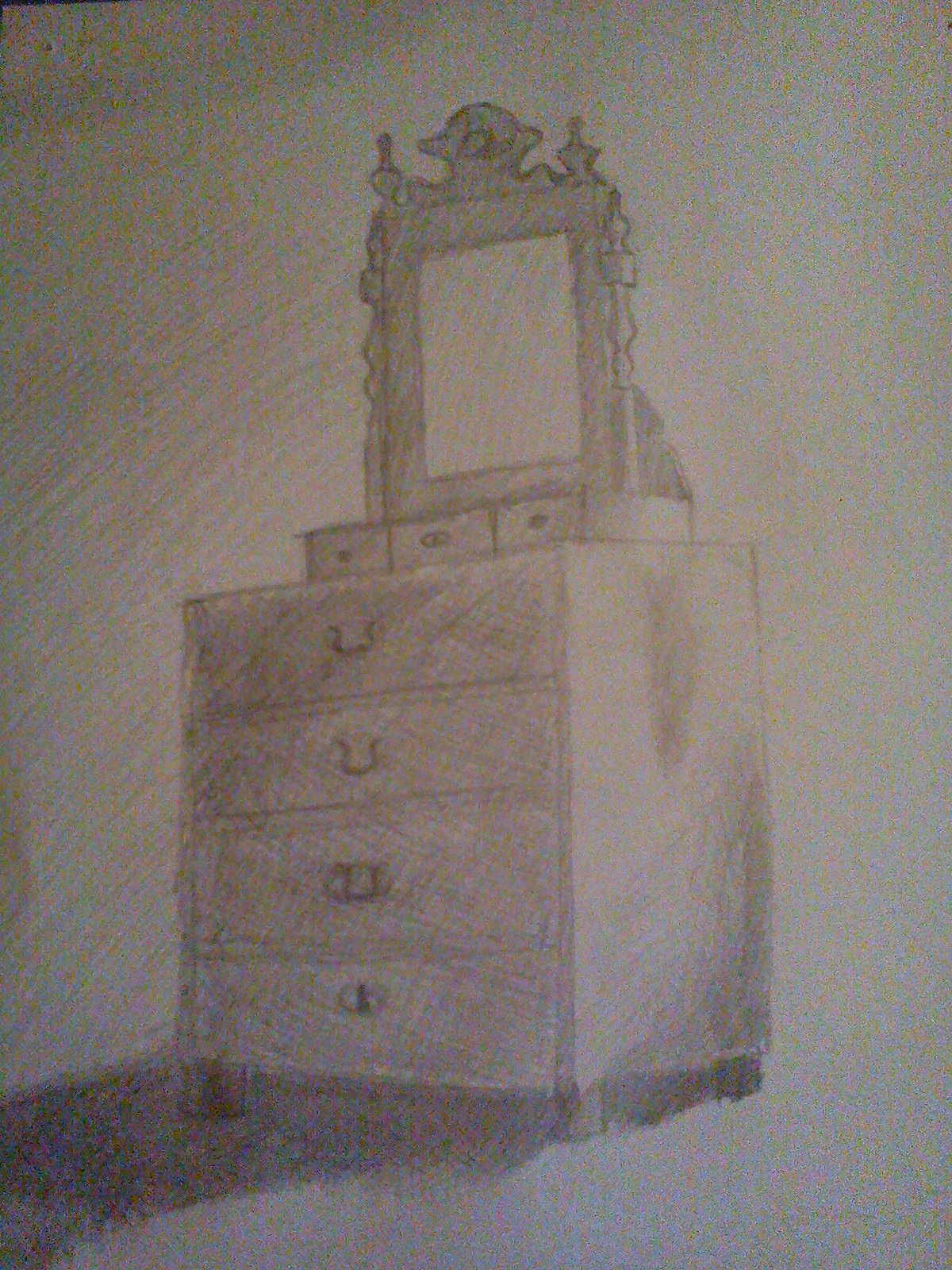A detailed pencil drawing depicts a high-standing dresser adorned with a vanity mirror. The dresser, rendered in black and white with meticulous line work, features four spacious drawers with metal handles that dangle invitingly, allowing easy access. The piece is crafted from plain wood and is richly detailed with an array of shading techniques, highlighting its depth and texture. A solid wood frame gracefully encircles the mirror above, and beneath it, two smaller "baby drawers" provide additional storage. The entire composition, captured from a low angle, emphasizes the dresser's imposing presence and showcases the artist's skillful use of shadows and pencil strokes.